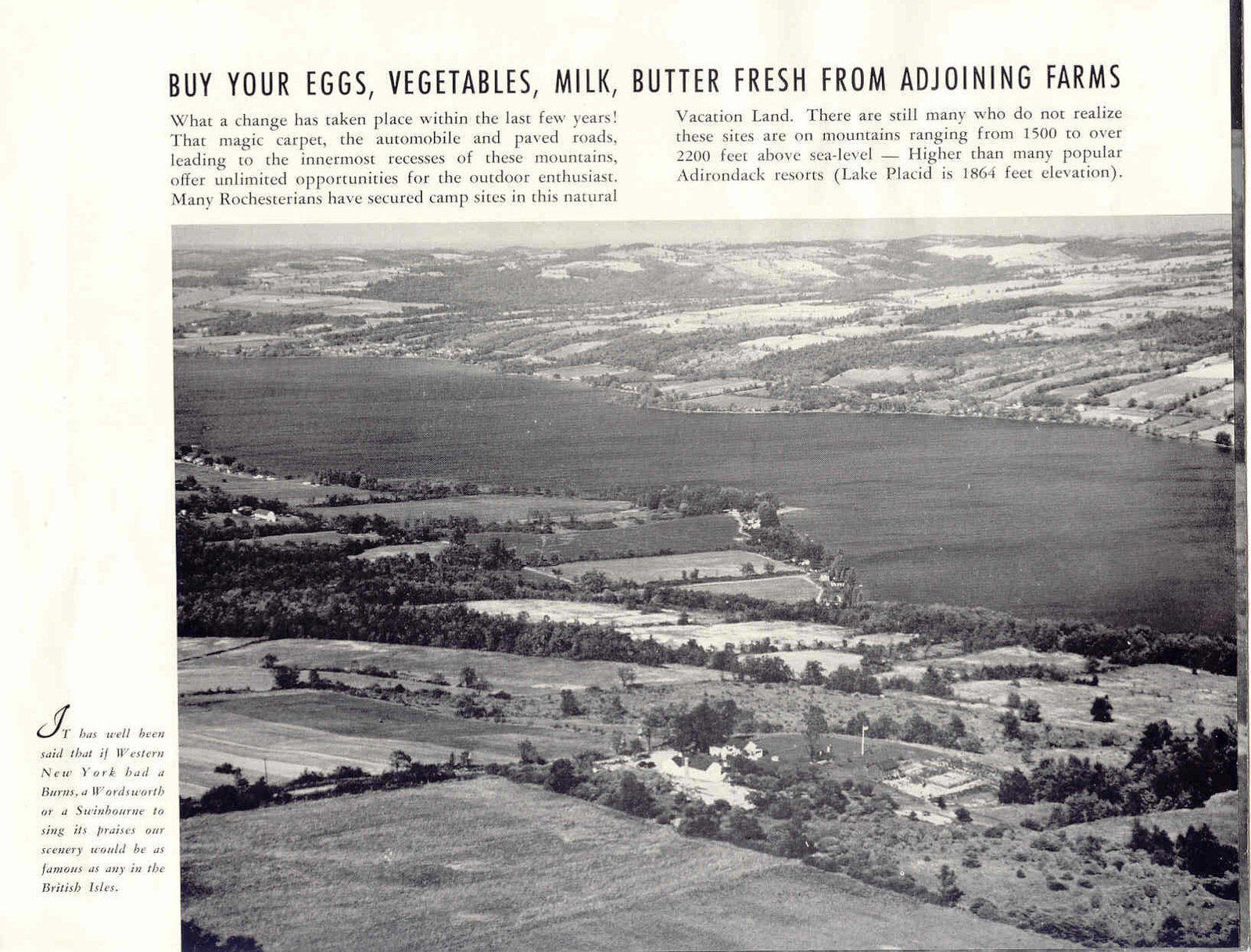Here's a detailed and cleaned-up descriptive caption for the image:

---

The image depicts a vintage newspaper or magazine clipping with a faded yellow background. At the top, the headline reads: "Buy Your Eggs, Vegetables, Milk, Water Fresh from Adjoining Farms." Below, the article comprises two paragraphs of text. The paragraph on the right begins with the statement, "What a change has taken place in the last few years. That magic carpet of the automobile and payroll is leading to the innermost recesses of these mountains, offering unlimited opportunities for the outdoor enthusiasts. Many Rochesterians have secured campsites in this natural vacation land." 

The paragraph on the left elaborates, stating, "There are still many who do not realize these sites are on mountains ranging from 1,500 to over 2,200 feet above sea level, higher than many popular Adirondack resorts. Lake Placid, for instance, is at 1,864 feet elevation."

Underneath the text, there is a large black-and-white photograph. It captures a serene river flowing through a verdant valley. The riverbanks are dotted with farms, outlined by lush green trees. The calm waters of the river have a gentle ripple effect. Beyond the river, rolling hills with sparse vegetation create a picturesque backdrop, predominantly white in color.

In the bottom left corner of the image, another paragraph reads, "It has been well said that if western New York had a Burns, a Wordsworth, or a Sundraus to laud its prairies, our sceneries would be as famous as any in the British Isles."

---

This caption provides a thorough and structured description of the image, bringing clarity and cohesion to the original spoken content.